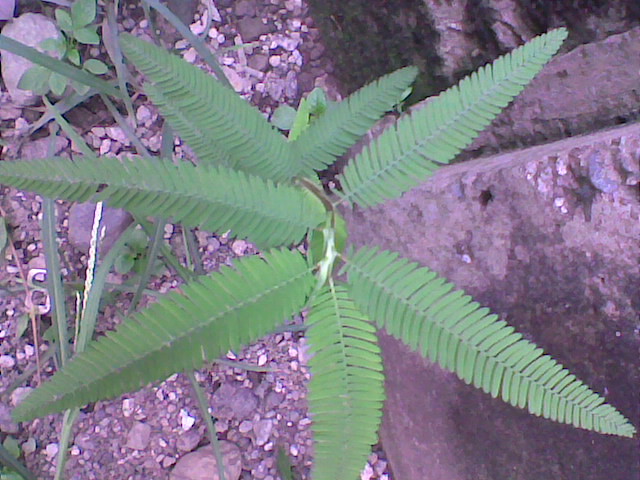In this image, we see a bird's-eye view of a lush, light green fern with seven fronds radiating outward like the spokes of a wheel. Each frond is adorned with finger-like leaves, converging at a central point in the heart of the plant. The fern is centered in a rocky terrain, where the ground is covered with purple and gray gravel interspersed with the occasional small weed and quack grass. Toward the bottom right of the frame lies a gray concrete slab, partially framed by the rocky surface that spans to the left. The overall setting suggests an urban or industrial area, possibly adjacent to a parking lot or amidst a cityscape. The photograph captures the rough, textured surface of the surrounding environment while focusing on the intricate details and vibrant color of the fern.